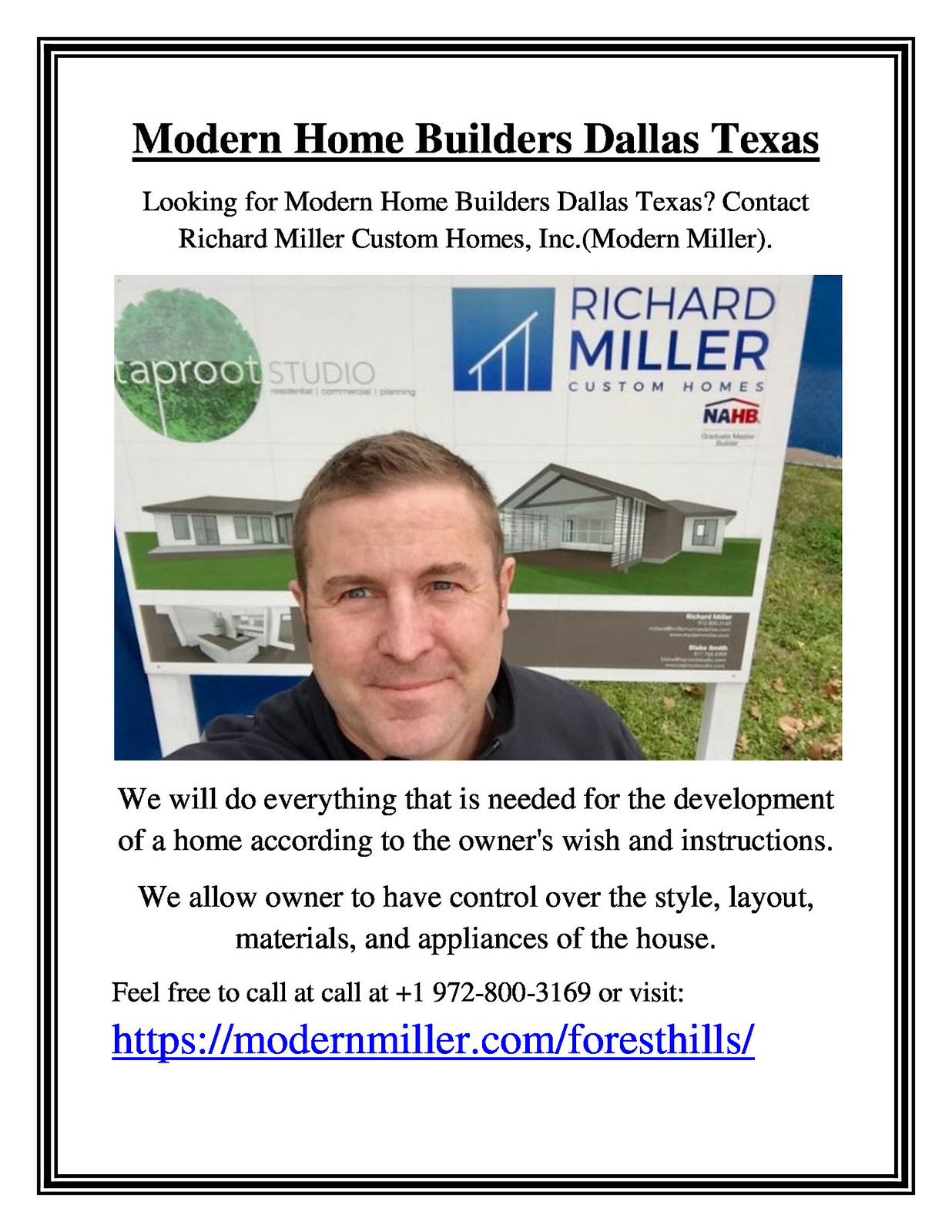The image is an advertisement with a prominent black frame and black text. At the top, bold and underlined, it reads "Modern Home Builders, Dallas, Texas." Directly beneath, it states, "Looking for Modern Home Builders, Dallas, Texas. Contact Richard Miller, Custom Homes Incorporated, Modern Miller." Featured prominently in the center is a photo of a smiling man standing in front of a sign displaying "Richard Miller" in blue text and "Taproot Studio" in gray against a white and green background, embellished with tree graphics within a green circle. This sign stands on green grass with brown leaves and is against a blue wall. The man, dressed in a dark-colored shirt, likely gray or black, stands before a housing structure marked by white siding and gray roofs. A key architectural feature includes a blue and red rooftop and a gray strip across the bottom of the sign. Below the photo, the advertisement states, "We will do everything that is needed for the development of a home according to the owner's wishes and instructions. We allow owners to have control over the style, layout, materials, and appliances of the house." Additionally, the contact details include a phone number, 1-972-800-3169, and a website, displayed in blue text: https://ModernMiller.com/ForestHills/.